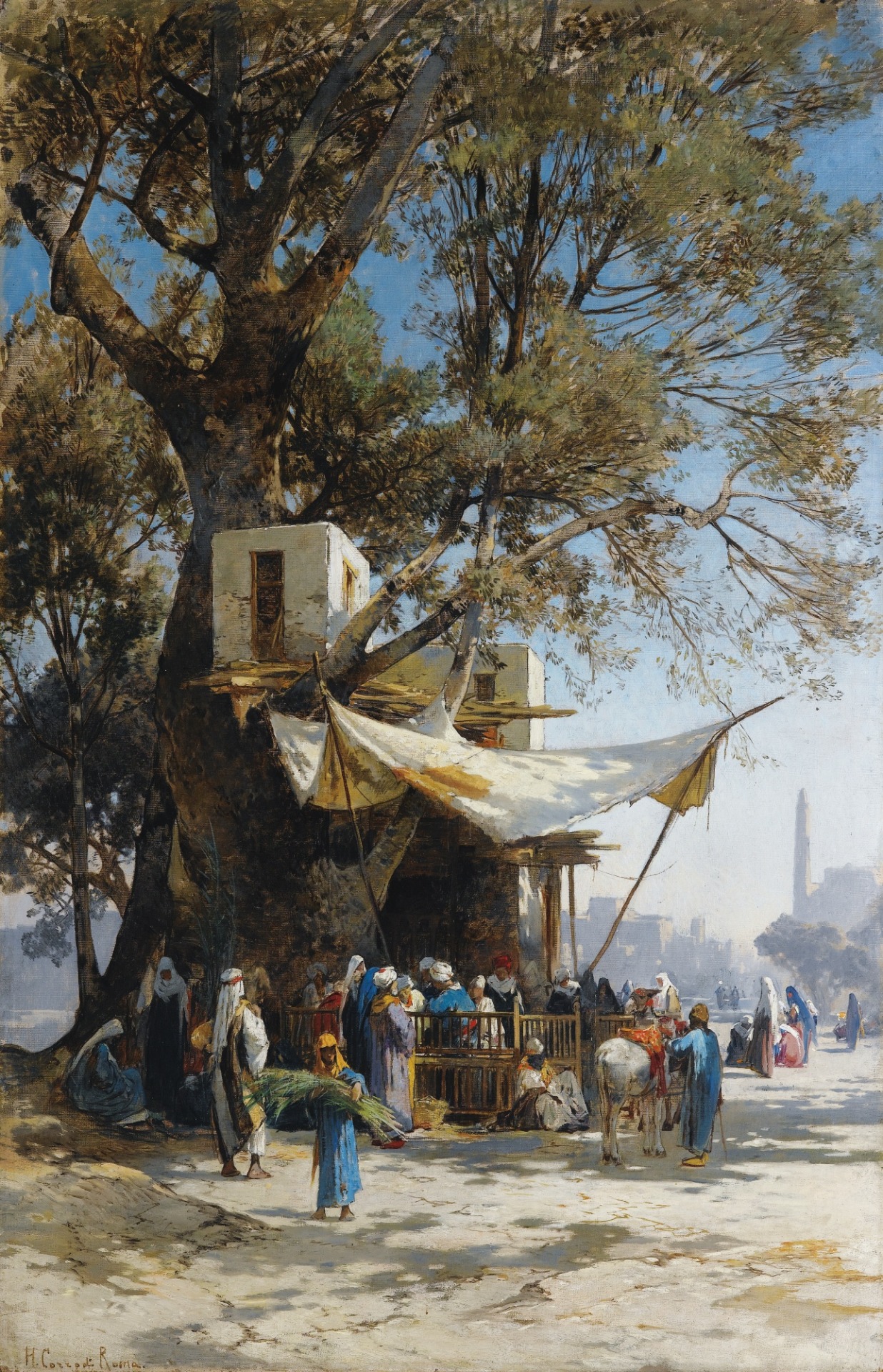This painting depicts a vibrant scene featuring a large crowd gathered around an enormous tree in what appears to be a Middle Eastern public area. The central focus is the tree itself, with its tall, dark trunk splitting into multiple substantial sub-trunks and branches. Draped from the tree is a large awning, possibly made of animal hide, supported by thin wooden posts. This awning shelters most of the individuals below. The people, numbering around twenty, are dressed in an array of colorful long robes in hues of blue, white, red, and black. Both men and women have their heads covered, some with turbans and others with loose fabric.

Central to the scene is the base of the tree, which incorporates building structures made of what appears to be white adobe or mud, featuring brown windows. A significant rectangular white building melds into the tree, reminiscent of a treehouse. A gold or brown gate encloses the area where people are standing.

In the foreground, a man leads a donkey adorned with an orange seat, suggesting provisions for someone to sit. The background reveals more of the bustling setting with some individuals moving toward and away from the central gathering. This area opens towards a roadway and extends into a distant cityscape, marked by modern buildings, a tall tower, and additional trees, all under a vibrant blue sky. The painting, despite its photorealistic detail, distinctly remains a masterful artwork.